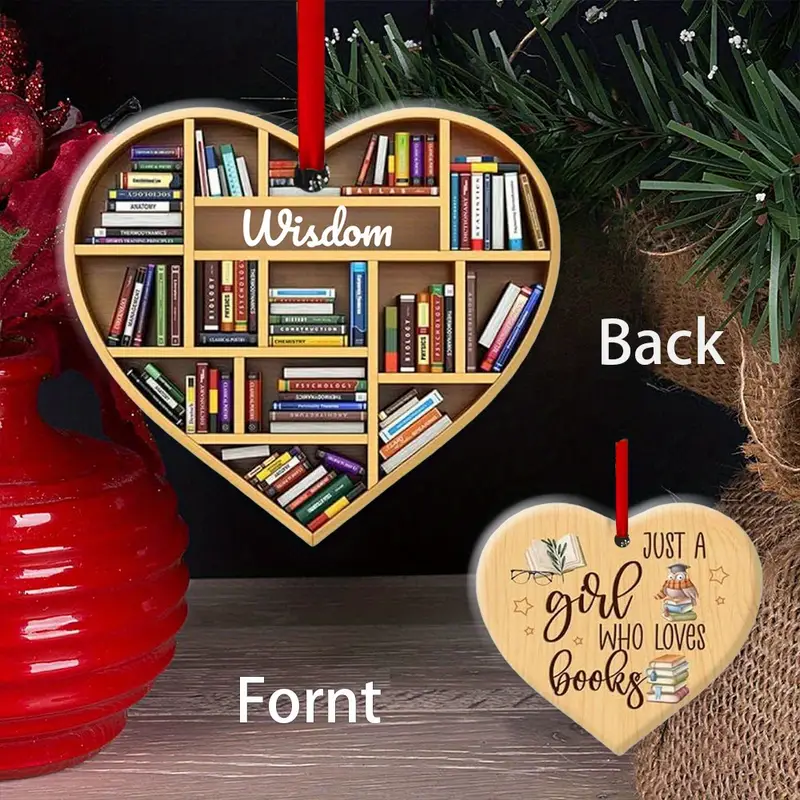In this image, we observe a heart-shaped Christmas ornament designed to resemble a bookshelf. The ornament is divided into shelves of various sizes and heights, with books stacked vertically, horizontally, and diagonally. One of the shelves prominently features the word "wisdom" in white script letters. The ornament is suspended by a red ribbon threaded through a hole at the top of the heart. Notably, there is a labeling error below the ornament, where the word "front" is misspelled as "F-O-R-N-T." The bottom right section of the image displays the back of the ornament, which showcases a design with books, an owl wearing a graduation cap and a scarf, stars, and reading glasses, accompanied by the phrase "just a girl who loves books." The background includes a tree wrapped in burlap and a red vase containing red and purple flowers.